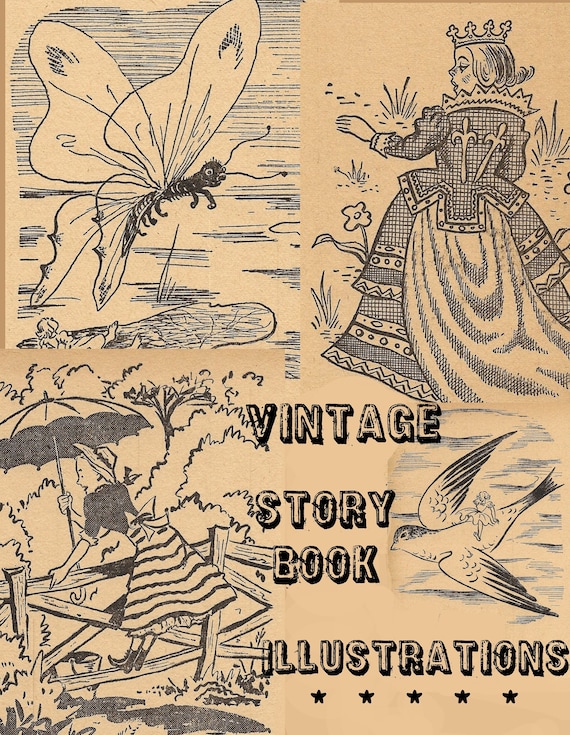The image showcases four intricate black pencil sketches on light brown, slightly yellowed paper, giving it an aged, vintage look. At the top left, a delicately drawn butterfly with long, black antennae and seemingly transparent wings appears to be in flight. On the top right, a regal queen is depicted from behind, adorned in a flowing, elaborate gown, with the left side of her face visible and a crown resting atop her head. The queen's detailed dress includes what seem to be two knife-like objects on her back. The bottom left features a woman in a skirt and hat, holding an umbrella, as she attempts to climb over a fence. Finally, at the bottom right, a bird (possibly a pigeon) is illustrated mid-flight, and on its back, a girl is seated. Near this sketch, the text reads "VINTAGE STORYBOOK ILLUSTRATIONS" accompanied by five black stars, emphasizing the nostalgic, storybook feel of the artwork.